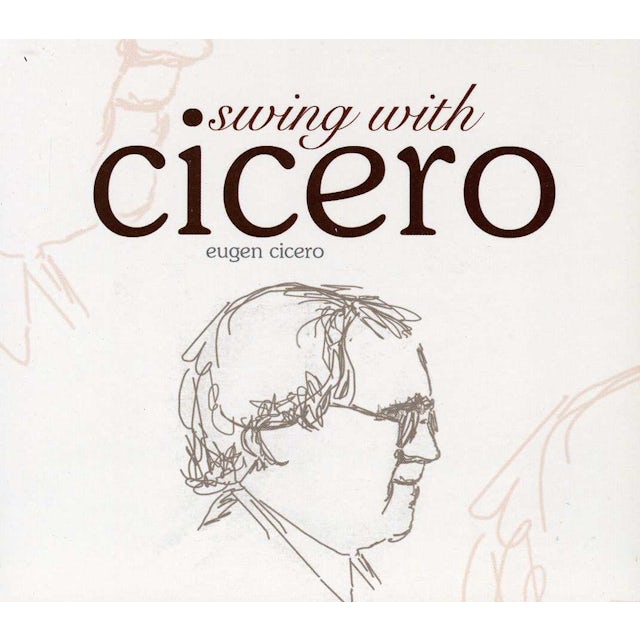The image appears to be the cover of a book or album with a tan background. In the upper left-hand corner, there is an abstract drawing in peach, possibly resembling the side view of a face from the nose down, although its exact shape is indeterminate. Central text in brown cursive reads "Swing with," followed by "Cicero" in large, dark brown letters. Below, in small gray letters, it says "Eugene Cicero." The illustration below the text is a black line sketch of a man's profile facing right. He has short hair, glasses, and wears a collared shirt. To the right of the sketch are abstract pink lines that form no clear shape. In the top left corner near the abstract drawing is another set of squiggly lines.